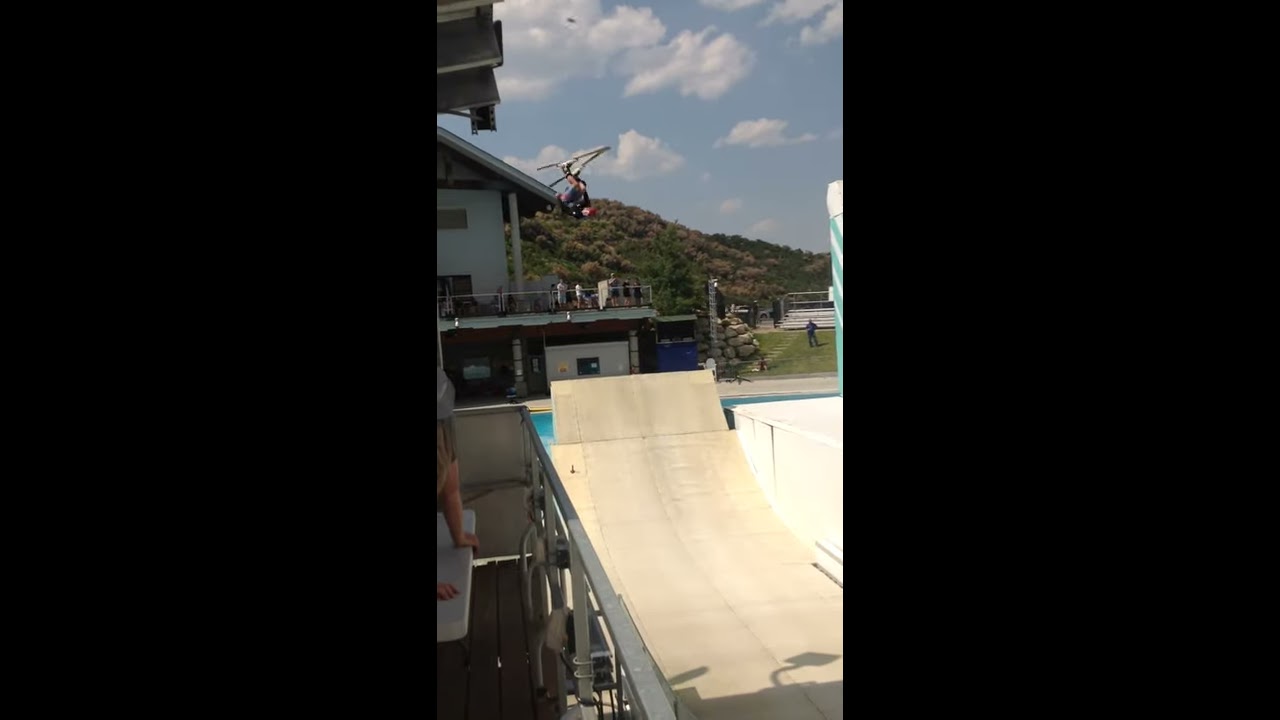The image features a vertically divided frame, with blacked-out sections on the left and right, focusing attention on the vibrant middle third. It depicts an outdoor scene showcasing a residential neighborhood set against slightly cloudy, but predominantly sunny blue skies. Puffy, cumulus clouds float above somewhat dry hills adorned with scattered shrubbery and low trees. Prominently, in the upper left-center, the image hints at either a modern windmill or helicopter blades against the backdrop of a hill.

In the foreground, a rectangular, white surface resembling a lounge chair or mat is apparent, possibly with wheels, placed on a deck made of light-washed wooden boards. To its left, the partial arms and the back of a person, possibly doing push-ups on a white mat, are visible. A house with a squared, boxy structure and a white façade is centrally featured, displaying multiple windows and a balcony that hints at a garage below. The right side of the house appears to have a rooftop garden or balcony with a grass-like area. In the upper center, an object suspended in the sky resembling a skier or stunt performer, adds an element of dynamic motion. The entire scene is both serene and active, combining elements of suburban stillness with subtle energetic nuances.